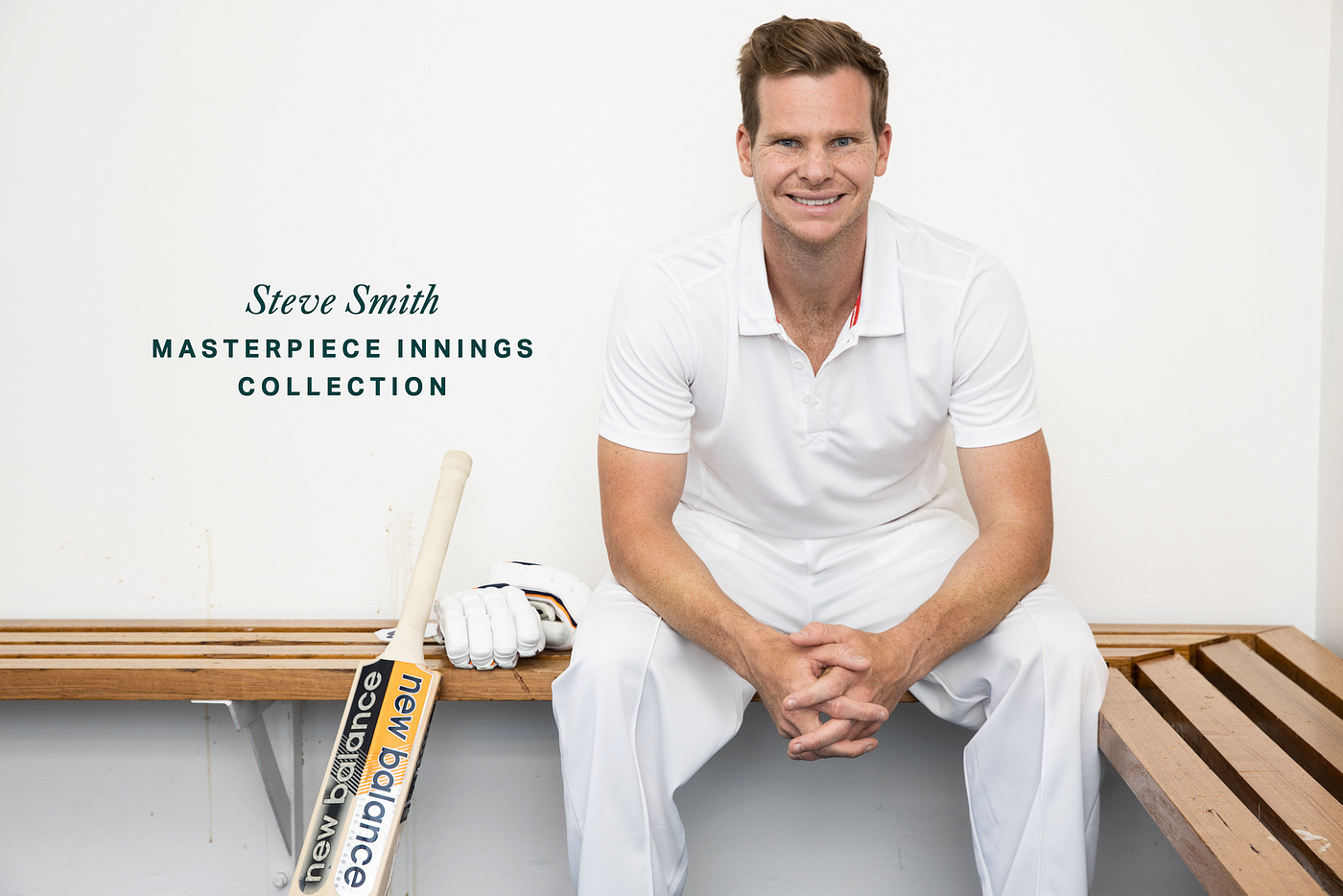In the image, a well-lit advertisement features a smiling white male, likely in his late 20s or early 30s, identified as Steve Smith. He has slicked-back brown hair, with a slight part on the left, and light blue eyes. Dressed in a white cricketer’s uniform, consisting of a short-sleeved polo shirt with an open collar and meticulously ironed white pants, he sits on a wooden bench composed of four slats that form a 90-degree angle. His elbows rest on his thighs, with his hands clasped together in front of him, highlighting his muscular arms. 

Behind him, a white wall serves as a neutral backdrop. To his left are a pair of white cricket gloves and a cricket bat, featuring the brand "New Balance" in white text on a black background. To the right of the writing, the firebrand name "New Balance" is also visible in black text on a yellow and white background. Above him, in stylized text, the name "Steve Smith" appears at a slight diagonal, with "MASTERPIECE INNINGS COLLECTION" in all capital letters below it. The setting suggests a sports advertisement focused on cricket gear, specifically endorsed by Steve Smith.